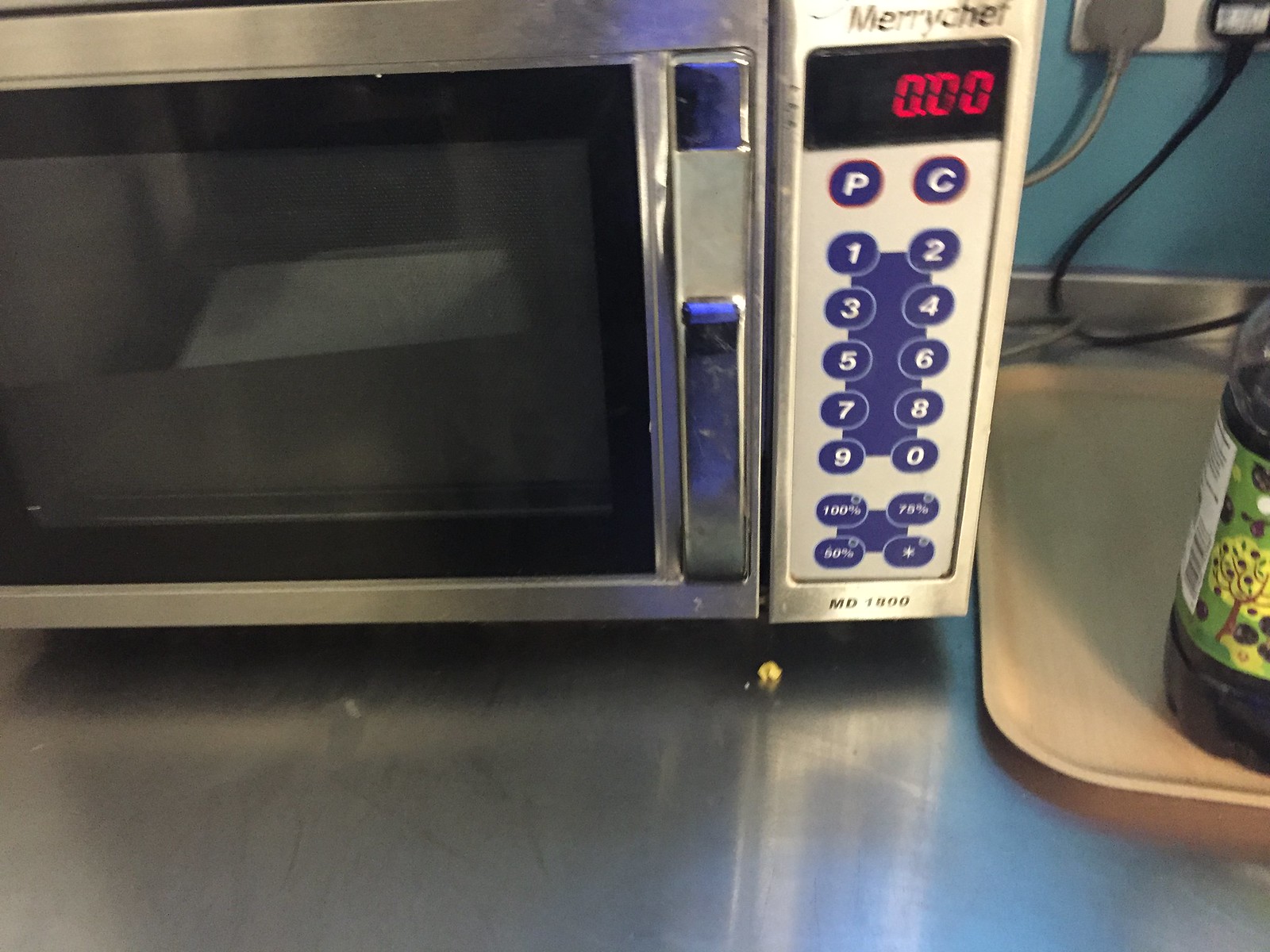In the photograph, there is a kitchen counter with a prominently placed vintage microwave that has a distinctly retro design, likely from the 1970s. This microwave, branded as "Mary Chef," features the brand name written in black lettering at the top right corner. The microwave has a metallic silver body with a matching silver handle and a black door that reflects a white surface. The handle appears to be broken but still functional. 

The control panel of the microwave is on the right side, showcasing an old-fashioned red digital display that currently shows "000." Below the display, there are two rows of circular blue buttons with white lettering and numbers. The first column consists of "P," followed by numbers 1, 3, 5, 7, and 9. The second column contains "C," followed by numbers 2, 4, 6, 8, and 0. Further below are buttons labeled "75%," an asterisk, "60%," "100%," and "MD 1800."

This microwave is placed on a silver-colored table where a small crumb is visible. To the right of the microwave, there is a wooden tray with a bottle, likely containing olive oil or a fruit-flavored drink, featuring a design with a tree and possibly blueberries. Additionally, two cords are plugged into an outlet on the wall behind the microwave.